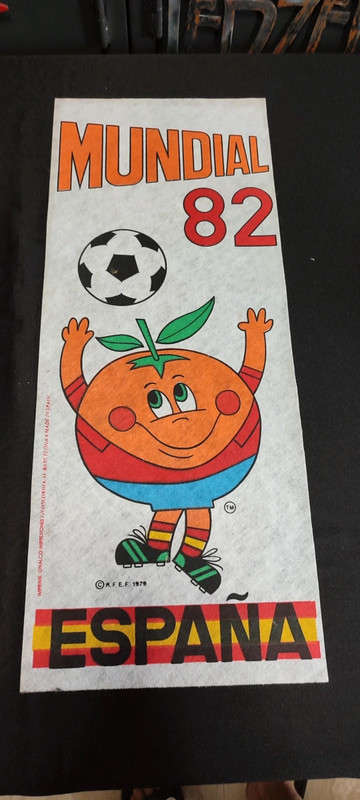The image features a rectangular, white poster or banner prominently displaying the text "Mundial 82" at the top. "Mundial" is written in all capitalized orange letters, while "82" is in red. Below this text is a black and white soccer ball in mid-air, with a cartoon orange character reaching up toward it, as if trying to catch it. The orange character is adorned with a red jersey, blue shorts, and red and yellow striped socks. It wears black soccer cleats with green stripes. The animated orange has green and black eyes, and its top features a green section resembling hair. Beneath the character, the word "España" is written in capitalized black letters set against a background that displays the red and yellow stripes of the Spanish flag. This detailed poster appears to be mounted on a high, black surface.